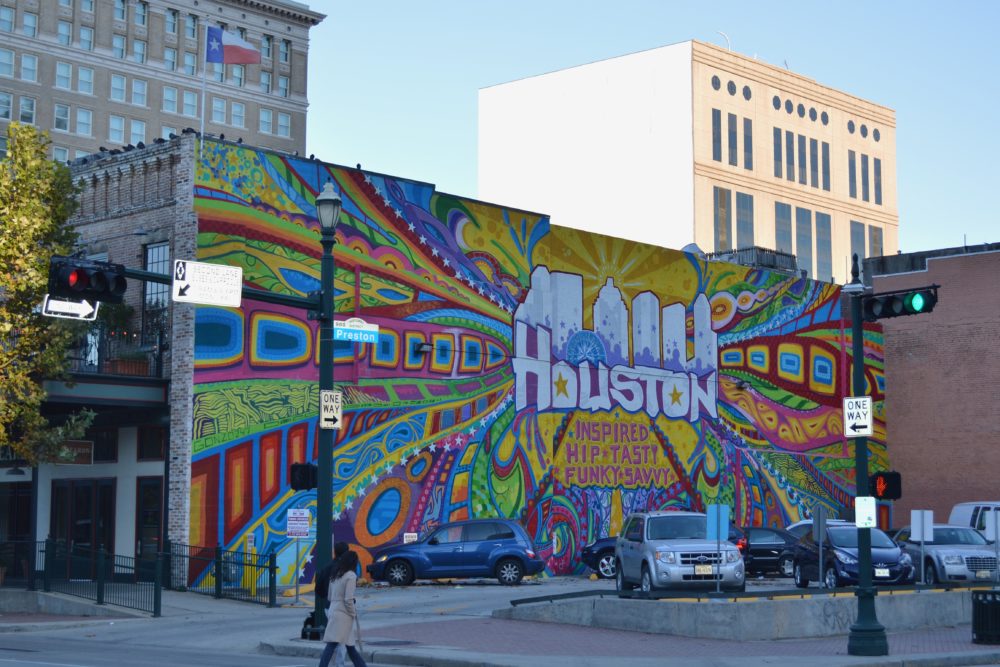This vibrant photograph captures a lively cityscape featuring a mural in Houston, Texas. The mural, located on the side of a foreground building, prominently showcases the word "Houston" with both O's designed as stars. The text is set against a colorful backdrop filled with psychedelic patterns of swirls, squares, and circles in a kaleidoscope of colors, including yellow, red, blue, green, pink, orange, and purple. The detailed artwork also includes a blue Ferris wheel and a white silhouette of the city's skyline, with stylized sun rays radiating around it. Accompanying the main Houston lettering are the words "Inspired, Hip, Tasty, Funky, Savvy", adding to the mural’s dynamic and funky aesthetic. Additionally, the image includes practical elements of the urban environment, such as parked cars in the foreground, a streetlight to the right, and a person crossing the street in the bottom left corner. The background features several large buildings, one of which proudly displays the Texas flag. This flag is distinct with its colors of yellow, red, blue, and a white star, further tying the artwork to its location.